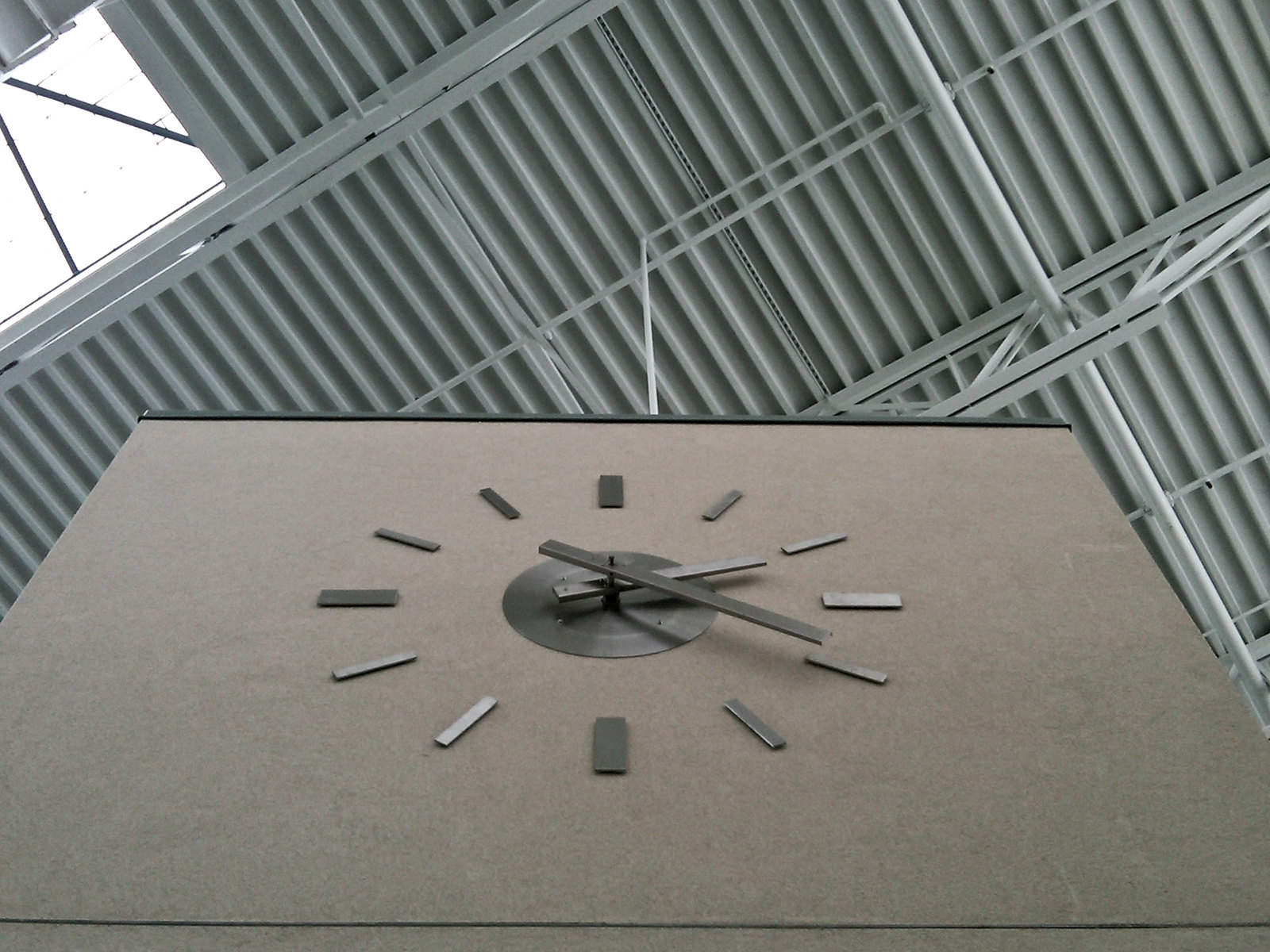The image captures a striking view of a minimalist clock mounted on a tall, brown wall, from a low perspective. The clock features simple, grey, square-shaped hands connected to a central pin, all mounted directly onto the wall. The numerals are represented by small, three-dimensional grey plates evenly spaced around the central point. Above the wall, the ceiling is visible with multiple rafters, and a small skylight is positioned to the far left. The scene is well-framed with the ceiling’s white lines in the background contrasting against the structured yet rustic appearance of the clock, giving an outdoor or industrial feel to the setting.